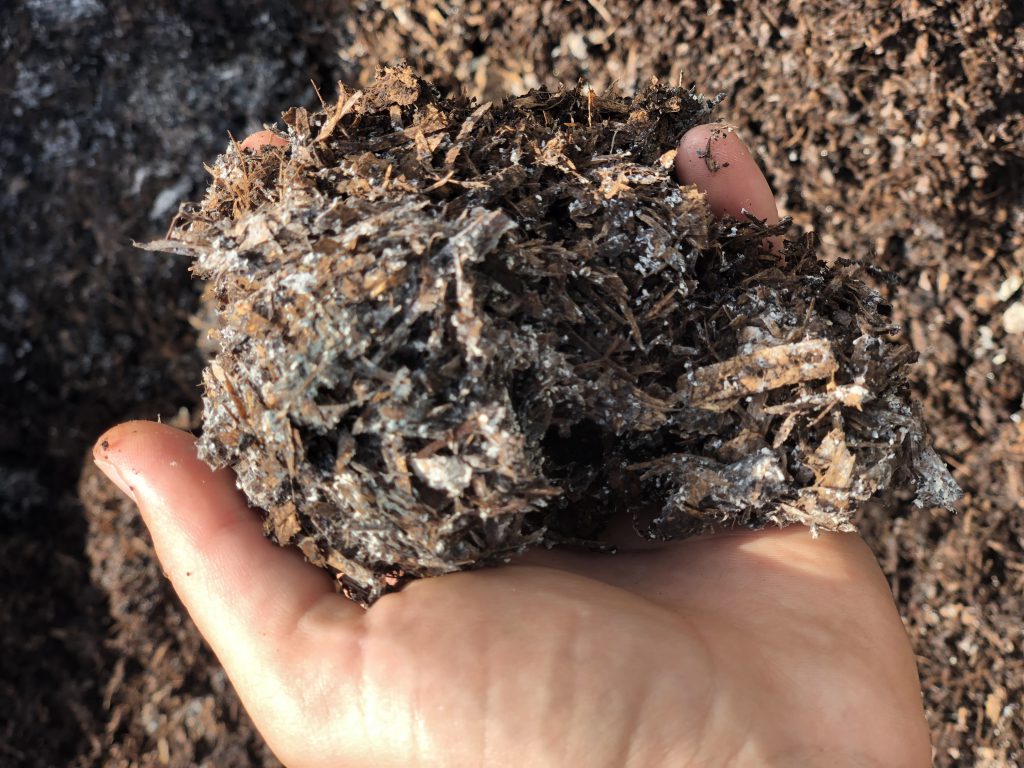The photograph captures a fair-skinned person's left hand, palm up, holding a clump of brownish mulch, which might be wood chips mixed with dried grass. Specks of white are scattered throughout the mulch, possibly indicating the presence of moss. The hand is largely clean, except for a bit of dirt on the fingertips. The background, though blurred, shows more of the same mulch-like material and suggests a sunny day with distinct areas of sunlit ground contrasted by shadow, hinting at an object or tree casting shade nearby.